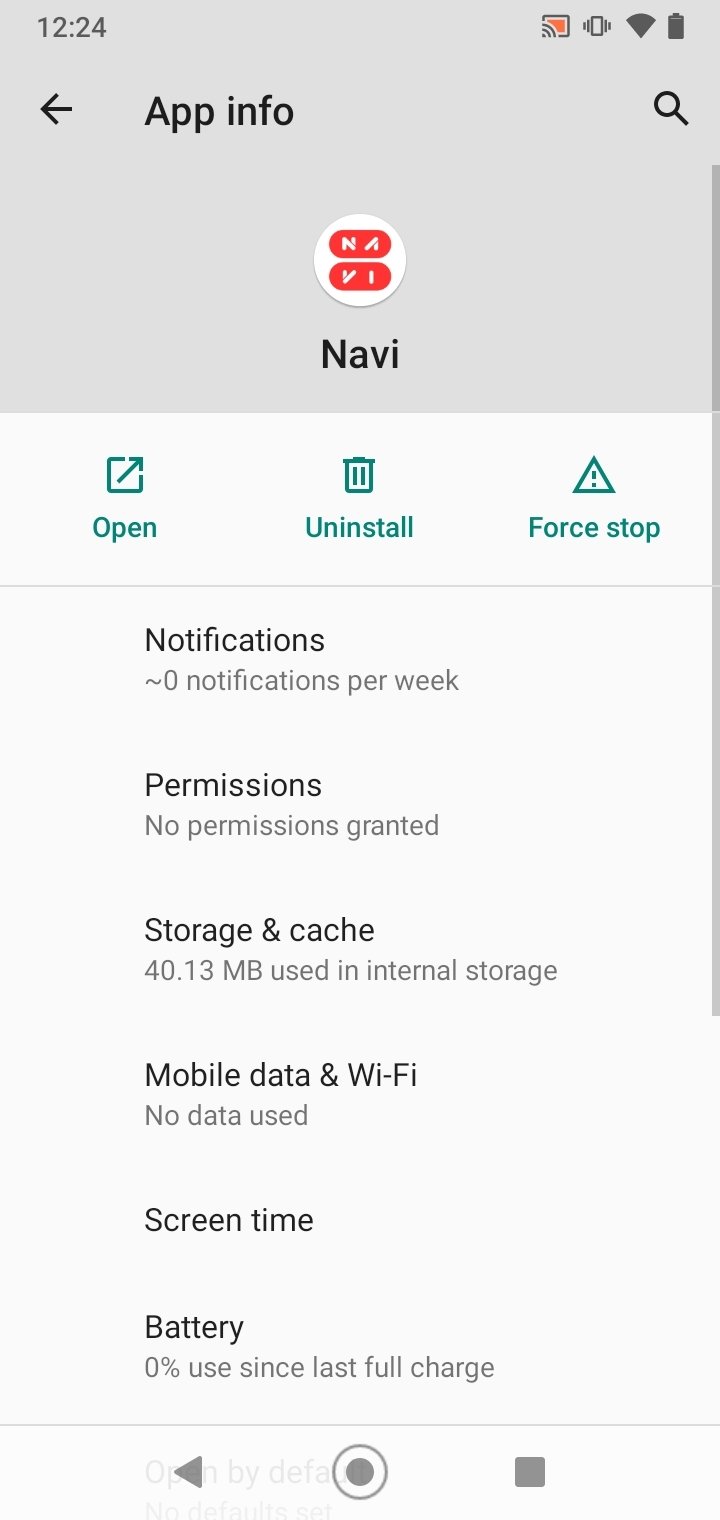This image showcases the App Info screen for an application named "Net Navy" on a smartphone. The screen displays various options and details about the app. At the top of the screen, the title "App Info" is prominently shown, followed by the app's name, "Net Navy." Below this, there are three actionable buttons: "Open," "Uninstall," and "Force Stop."

Further down, a series of categories are listed with brief information:
- **Notifications**
- **Permissions**
- **Storage and Cache**
- **Mobile Data & Wi-Fi**, which states "No Data Used."
- **Screen Time**
- **Battery**, indicating "0% used since last charge."

At the bottom of the screen, three navigation icons are visible: a sideways triangle (likely for back), a circle within a circle (home), and a square (recent apps). Additionally, the top portion of the screen features status bar icons including the time "12:24," Wi-Fi, battery, and casting icons.